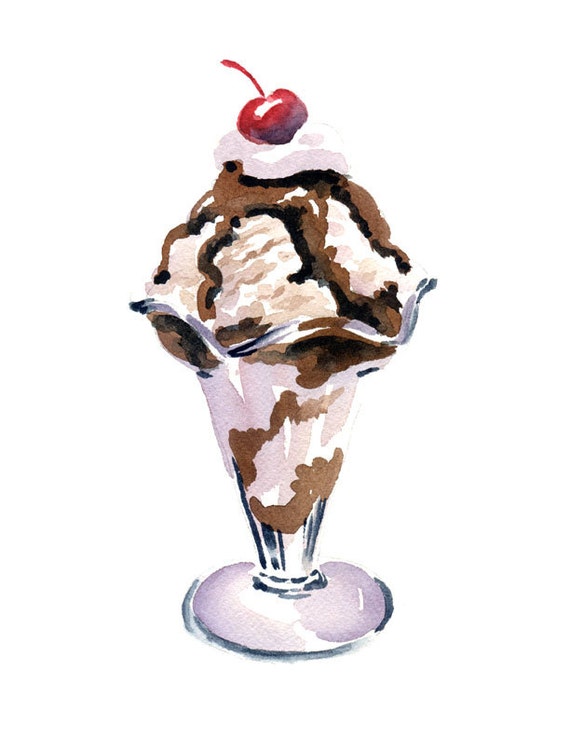The image is a simple, artistic watercolor painting of an ice cream sundae, centered against a pure white background. It features a single, transparent glass bowl with a circular base that tapers to a point at the bottom and broadens into a curved, wave-like pattern along the top edge. The sundae comprises layers of vanilla ice cream with chocolate highlights on the bottom, more vanilla ice cream with chocolate drizzle throughout, and finally, a generous dollop of whipped cream topped with a cherry stem. The glass container showcases pale blue hues with darker navy blue and black shading for depth and interest, particularly in the areas depicting the fudge. The overall depiction showcases subtle watercolor effects, giving a sense of delicacy and artistic allure, making it look appetizing despite being a painting.